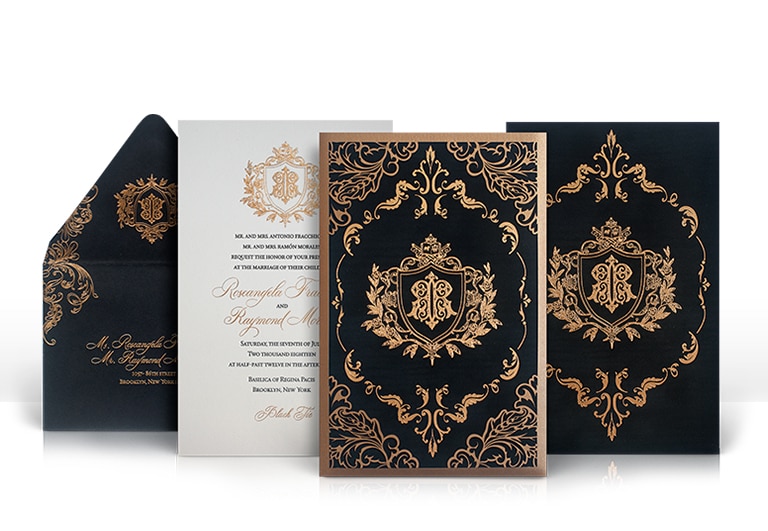This image showcases an elegant set of invitations presented against a pristine white background. On the left, there is a partially open black envelope adorned with intricate bronze-gold filigree. The envelope seems to hold a white piece of paper, which is the main invitation. The invitation features an opulent gold shield at the top, surrounded by delicate filigree, and includes black text detailing the event's specifics. In the center, two names are rendered in graceful gold script, with a block of text below that provides the date and further details in black. At the bottom center, "black tie" is prominently displayed in gold lettering. To the right of the invitation, there's another black piece of paper featuring a gold border and extensive filigree that mirrors the ornate design of the envelope. Adjacent to this, the same black piece appears again, this time without a border, resplendent with gold decorations. The overall presentation exudes a regal and sophisticated air, suggesting an exclusive and formal event.